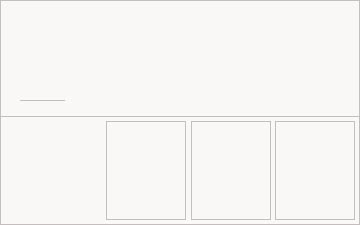Caption: "This is a minimalist screenshot of a website's layout featuring an off-white background with outlined sections. The top portion of the image displays a horizontally elongated rectangle with a small line in the lower left corner, but otherwise remains empty. Below this, the screenshot is divided into another rectangle that contains three outlined squares aligned from right to left. The sequence starts with three empty square outlines, followed by a blank space where another square could fit but is not outlined. The image overall highlights the skeletal structure of the web design, devoid of any actual content."